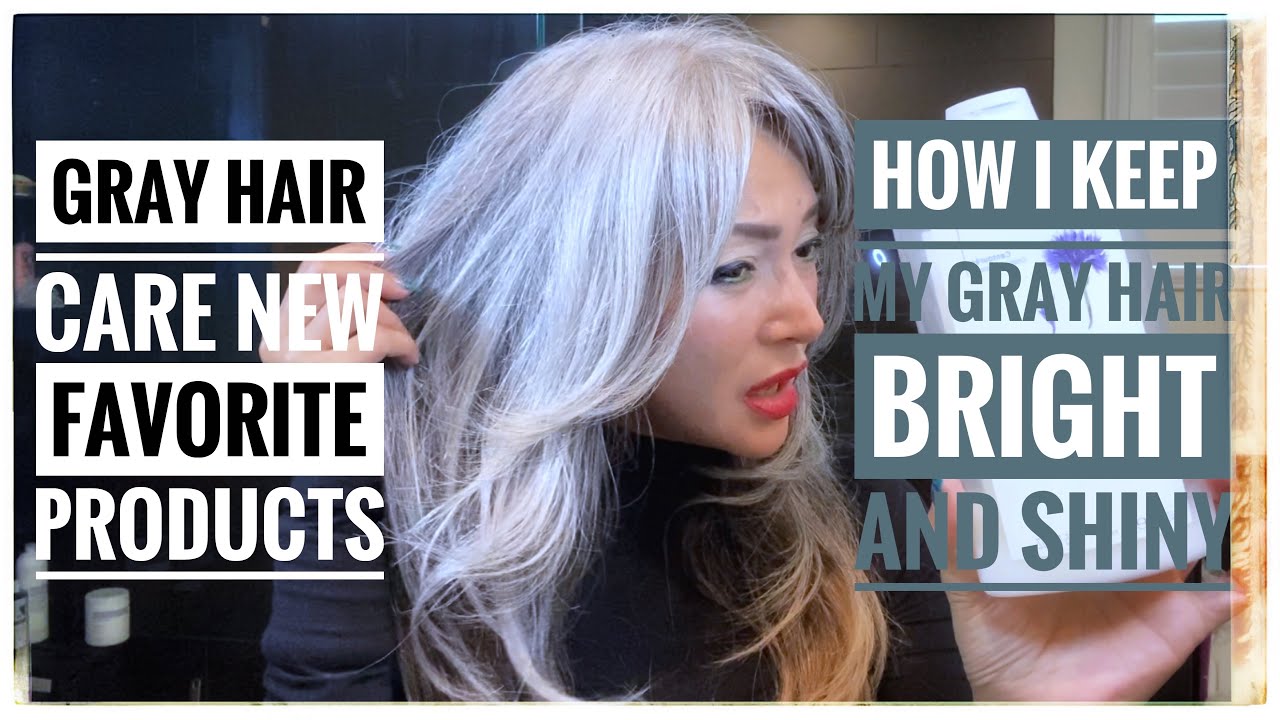In the image, a woman with light skin, dark eyes, and striking red lips is posing in front of the camera. Her body is fully facing forward, but her head is turned three-quarters to her left, allowing a detailed view of her elegant profile. She has long, gray hair that cascades down to her chest, and she is delicately picking up a section of her hair with her right hand. In her left hand, she holds up a white bottle adorned with a blue design, presenting it to the camera. The bottle's details are somewhat obscured by overlaid text. The text on the left side of the photo reads, "Gray Hair Care: New Favorite Products," while on the right side, it states, "How I Keep My Gray Hair Bright and Shiny." The image captures the woman proudly showcasing her hair care product amidst the informative and inviting text.